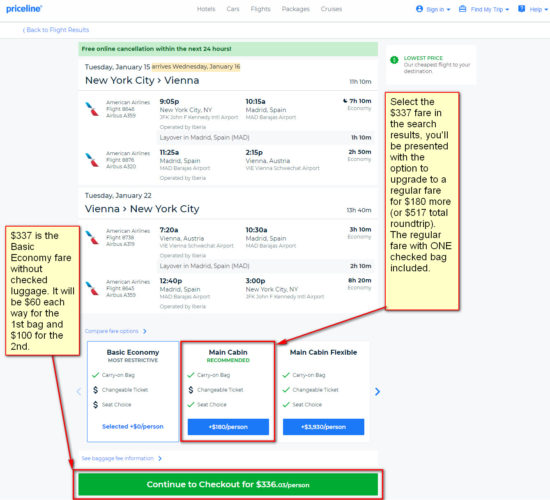This image is a detailed screenshot from Priceline, a travel booking website. The page features a clean, white background with a matching white header. In the upper left corner, the Priceline logo is displayed in blue, lowercase letters. The central part of the header contains a gray menu with options listed as: Hotels, Cars, Flights, Packages, and Cruises. On the right side, the blue font labels include "Sign In" and other smaller, unreadable items.

In the main section of the screenshot, a flight search is displayed. The selected route is New York City to Vienna, highlighted in dark gray font, with the departure date set for Tuesday, January 15th. Specific flight departure and arrival times are indicated but are too small to read. The return flight from Vienna to New York City is set for Tuesday, January 2nd, again with unreadable times.

On the right side, a prominent long vertical rectangle with a light yellow background and red outline contains important fare information. In black font, it instructs users to "select the $337 fare in the search results. You'll be presented with the option to upgrade to a regular fare for $180 more or $517 total round trip," with the regular fare including one checked bag.

On the left side, another rectangle, smaller in size, provides additional fare details. It states that "$337 is the basic economy fare without checked luggage. It will be $60 each way for the first bag and $100 for the second."

At the bottom of the page, a green rectangle with white font directs users to "continue to checkout for $336."